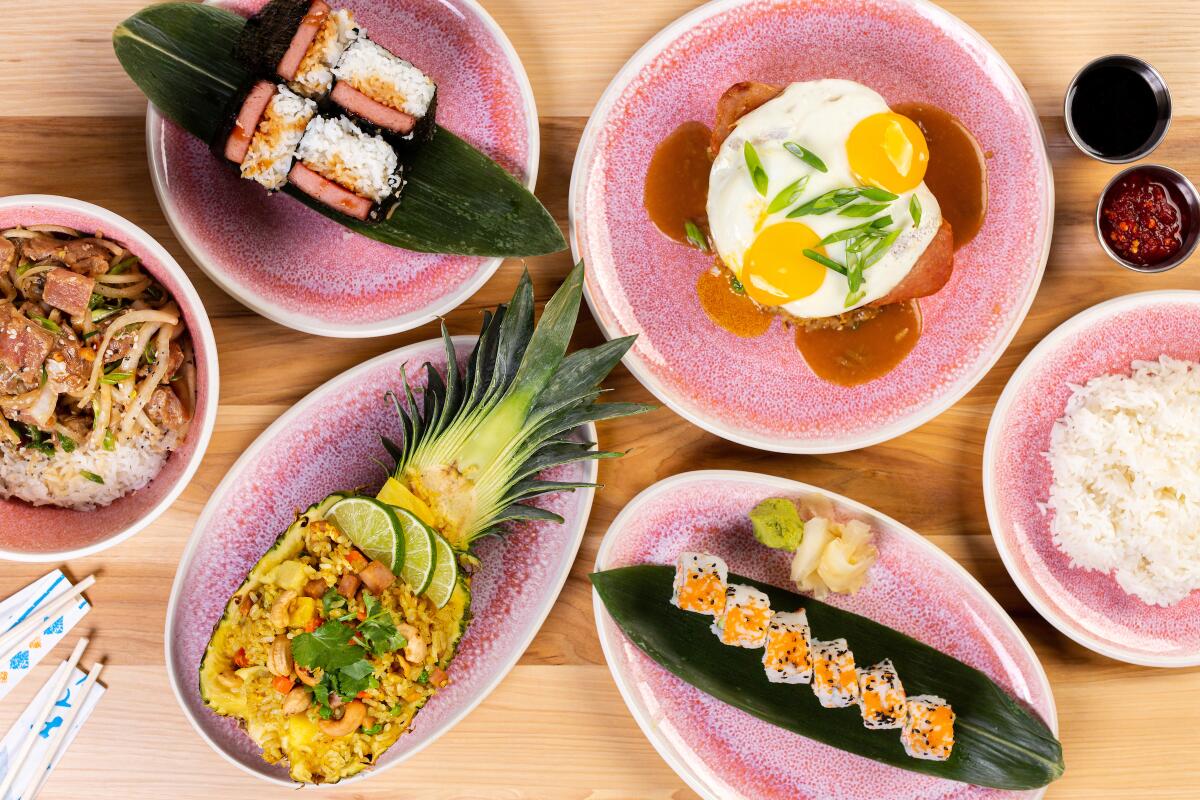The image depicts a vibrant assortment of culinary delights meticulously arranged on a light-colored wooden table. There are six dishes in total, each set in pink bowls and plates adorned with white rims. Starting from the bottom left, there are two sets of chopsticks and a bowl containing a mix of rice, meat, and vegetables. Moving clockwise, the next plate features a green leaf topped with four square pieces of sushi. Adjacent to that is a dish with two sunny-side-up eggs, garnished with greens and a brown sauce. 

In the upper right corner, two small metal containers hold soy sauce and a red chili sauce, respectively. Below them is a bowl of plain white rice. Continuing clockwise, the bottom right plate features another green leaf with six cubes of sushi, interspersed with a few small, indeterminate fruits. Finally, on the left side, an oval plate presents a pineapple cut in half, stuffed with limes, additional garnishes, and possibly chunks of meat. The overall scene suggests a feast inspired by Asian cuisine, elegantly presented on a wooden table with varying shades of brown.